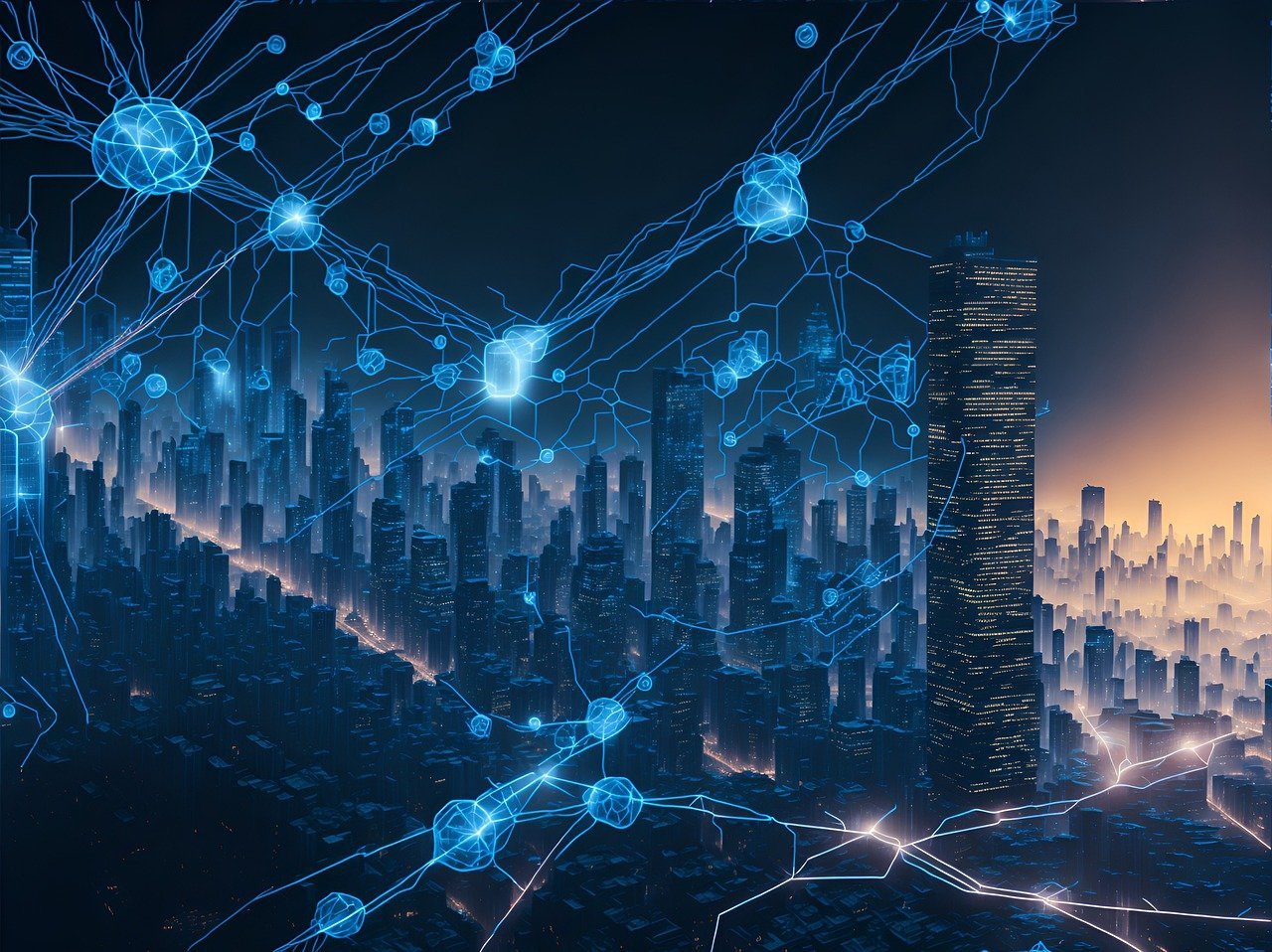The image is a digital, artistic, and sci-fi depiction of a sprawling city skyline viewed from above at dusk. Towering skyscrapers dominate the scene, with the buildings in the foreground brightly illuminated by numerous lights, while those in the background blend into the darkened sky. To the left, a nearly setting sun casts a yellowish foggy haze over the city, adding a dramatic effect. Blue, glowing blots connected by thin, electric-like lines intermingle throughout the cityscape, resembling electricity pulsing in the air. These blue shapes, somewhat like jellyfish, float above the city, creating an otherworldly and interconnected network of luminous energy. Additionally, a yellowish line toward the upper left resembles traffic lights or cars moving through a surreal, energy-laden roadway.